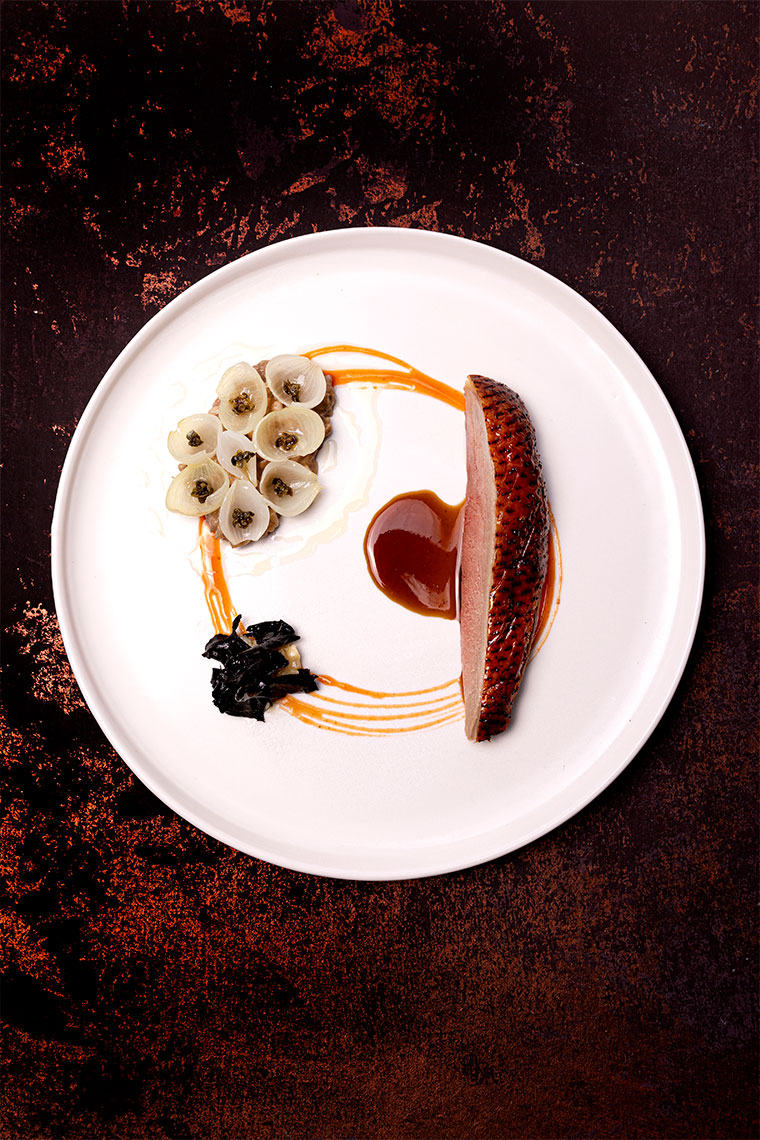The image depicts a meticulously arranged dish on a round white plate, set against a striking red and black background. Dominating the right side of the plate, there's a long piece of sliced meat, featuring a visually intriguing combination of pale red and white flesh, with a boar-skin-like dark red and black crust, flecked with spots. This protein is drizzled underneath with a rich, dark red sauce. In the center of the plate, a vibrant orange sauce is swirled artistically, creating a focal point. At the top left, a cluster of tiny, open clamshells are presented, each holding small brown and black spheres, possibly caviar. Nestled below the shell cluster is a delicate leafy green. The bottom left of the plate features a mysterious pile of black, crumpled paper-like substance. The artistic arrangement and variation of textures and colors make the dish both a culinary and visual masterpiece.